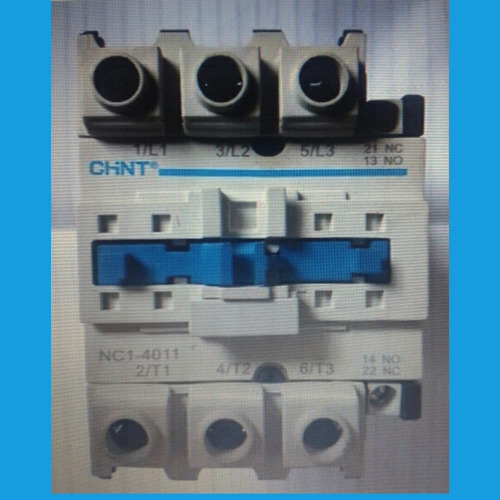The image depicts a piece of scientific or electrical equipment placed against a light blue background, possibly on top of printer paper. The equipment is characterized by a white plastic surface with prominent features. At the top and bottom of the structure, there are three tower-like shapes, each housing a circular opening—these may function as input connectors, possibly for hoses or cables. 

Labeling on the top three openings includes numbers and letters: from left to right, 1-L1, 3-L2, and 5-L3. Centrally located is a rectangular area filled with smaller square cutouts that surround a larger blue rectangular component. This piece features the blue letters "CHNT" on the upper left beside a horizontal blue bar stretching across. The overall impression is that this apparatus is designed for connectivity and control within an electrical or networking system.